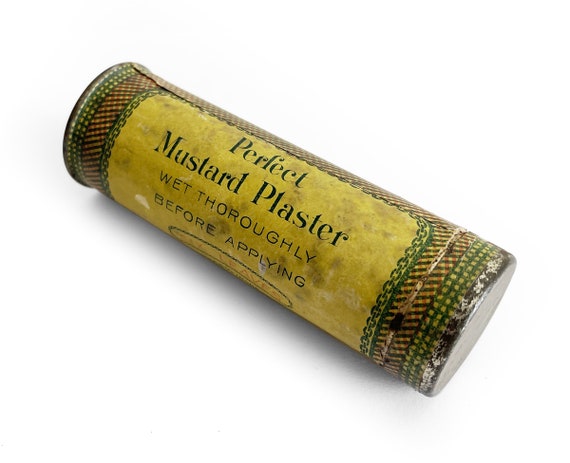The photograph features a cylindrical, vintage metal canister set against a white background, tilted at a 45-degree angle, with the left end pointing toward the top left corner and the right end toward the bottom right. The canister, clearly showing its age with multiple stains, dents, and signs of wear, has a label in the center bordered by a green chain-like design on a heavily stained yellow background. The label's black text reads: "Perfect Mustard Plaster. Wet thoroughly before applying." Surrounding the main label is an intricate arrangement of patterns—a green and white checkered border around the cylindrical ends, a red, black, and white plaid section closer to the center, and an orange-and-black checkered pattern further out. The container also displays areas with brownish-yellow discoloration and additional white spots, emphasizing its extreme age and vintage condition.